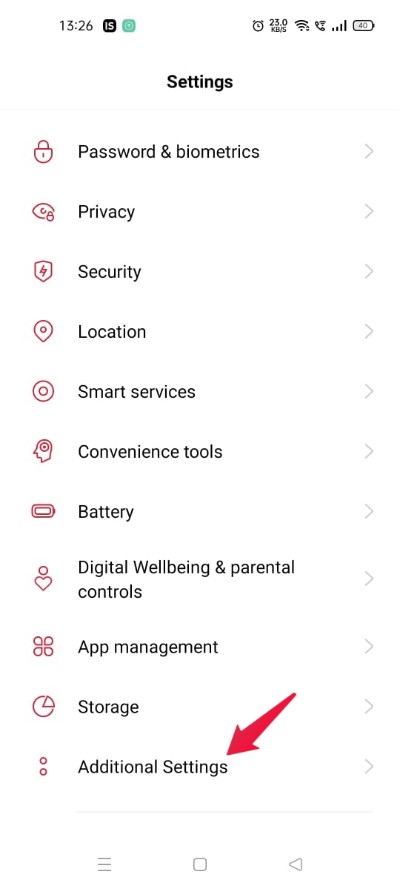**Screenshot Description: Detailed View of Phone Settings Menu**

The screenshot depicts a phone screen captured at 13:26, as indicated by the time in the upper left corner. The device's battery level is at 40%, shown in the upper right corner. Dominating the top section of the screen is the word "Settings," prominently displayed in bold black text. Below this, a thin gray line separates the heading from a comprehensive menu of settings options.

The menu is organized in a column with icons and text, facilitating navigation through various settings. The icons are uniformly red and positioned on the leftmost side of the column, accompanied by descriptive text and a right-facing arrow indicating sub-menu access. The options are listed in the following order from top to bottom:

1. Password and Biometrics
2. Privacy
3. Security
4. Location
5. Smart Services
6. Convenience Tools
7. Battery
8. Digital Well-being and Parental Controls
9. App Management
10. Storage
11. Additional Settings

A large, noticeable red arrow points directly to the "Additional Settings" text, drawing attention to this specific menu option. This arrow suggests an emphasis or a prompt to explore further within the "Additional Settings" category.